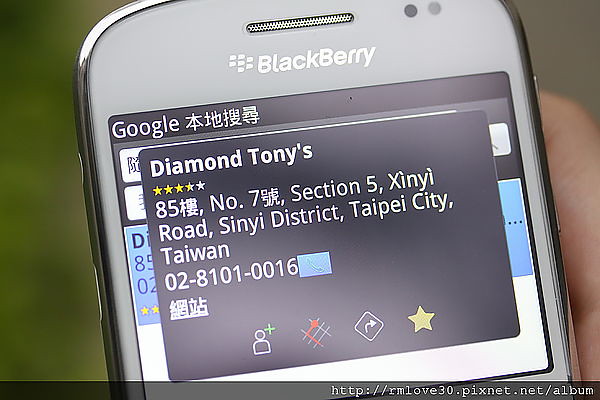The image captures a close-up of a person holding and photographing the screen of an old flip-out BlackBerry phone, identifiable by the "BlackBerry" label in white on the top of its green-grey casing, with seven dots adjacent to it on the left. The phone's display is rectangular and currently shows a mix of text and icons. At the top of the screen, the word "Google" is prominently displayed, accompanied by Chinese characters. Below it, a black dialogue box contains the notification "Diamond Tonys," followed by a star rating featuring three and a half golden stars. The information beneath this includes the address: "Section 5, Xinyi Road, Xinyi District, Taipei City, Taiwan," and the contact number "02-8101-0016" with a call icon next to it. The bottom of the screen displays various icons, including a follower icon, a hashtag icon, a directional icon, and a yellow star icon, all arranged horizontally. The background of the image is blurred but shows a person’s finger holding the phone on the right side and a green hue, possibly foliage, on the left. There is also a printed URL at the bottom right, "http://rmlove30.pixnet.net.album," in white text. The overall composition is a blend of photographic representational realism.